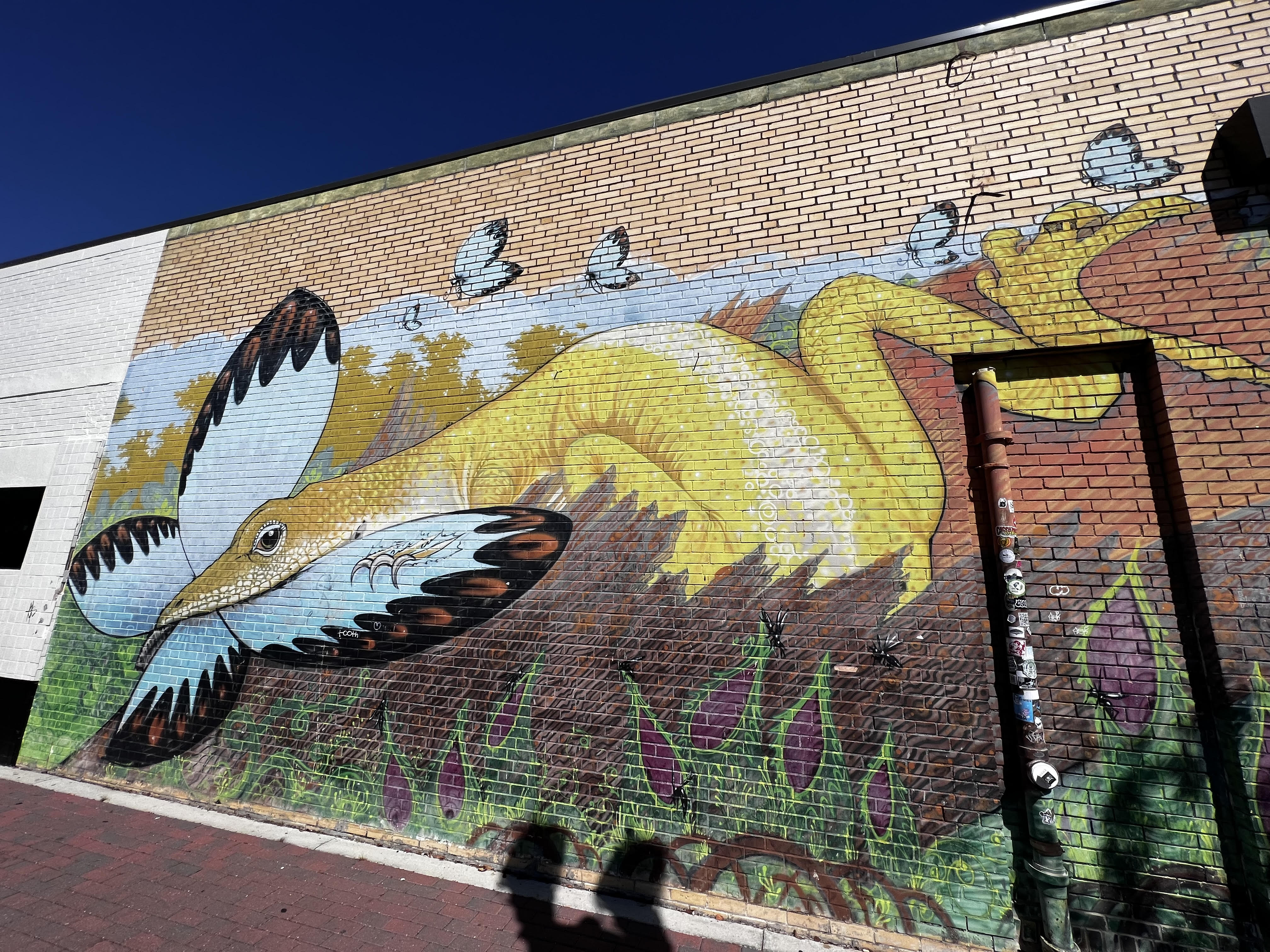This is a daylight photograph of a vibrant graffiti mural on the side of a brick building, captured at an angle that makes it appear as if the building is leaning backwards at the top. The mural occupies most of the right side of the image and narrows as it moves leftward. At the bottom of the photograph, there's a shadow cast by a parking meter on a brick-colored sidewalk.

The mural vividly depicts a woodland scene featuring a large, pale yellow lizard with a stripe along its back, clutching and consuming a large butterfly. The butterfly, located in the lower left corner, has blue wings with brown tips. The lizard's sharp claws are seen tearing into the butterfly's wings, while its mouth engulfs the body. Above this scene, four smaller butterflies, white and brown, are fluttering across a sandstone-colored section of the brick wall.

At the bottom of the mural, the ground is depicted with dark brown and green grass, interspersed with indistinct purple and green pitcher plants that have small insects around them. The mural doesn't entirely cover the wall; portions of the natural brick are visible at the top. In the top left corner of the image, a deep blue sky is evident. There’s also a service pipe painted over by the mural at the lower right side, providing access to the building's interior. The mural, blending vibrant and natural colors, portrays the lizard in a dramatic moment within its forest-like habitat.